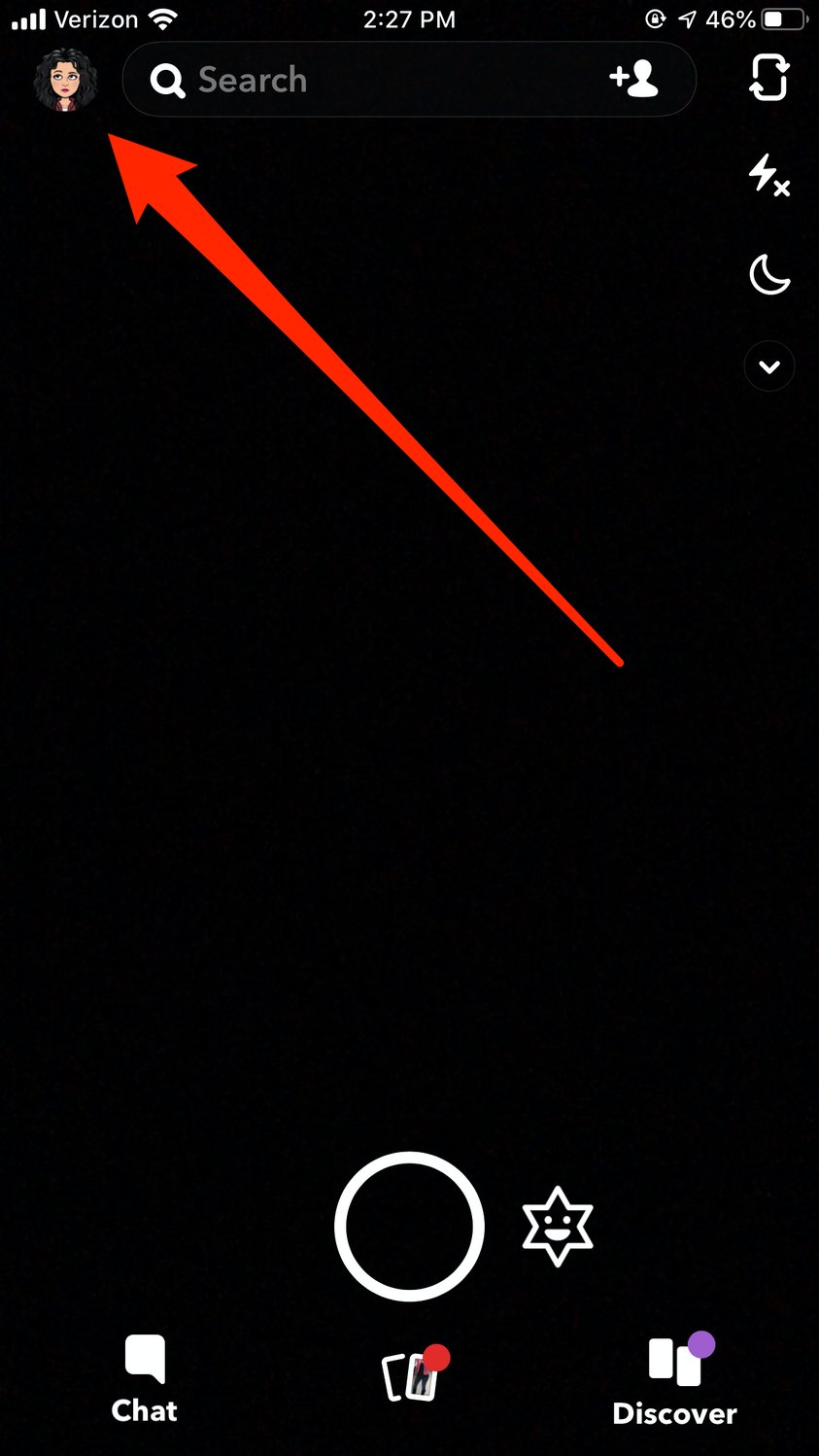The image depicts a screenshot of an unidentified chat application on a tablet. The background is entirely black, providing a stark contrast to the predominantly white elements displayed. In the upper right corner, standard tablet interface icons are visible, including a battery indicator showing 46% with no charging symbol, a plus sign next to a small white figure icon for adding users, and the usual battery and Wi-Fi icons. 

On the upper left, there is a search bar, the Verizon symbol, and a small avatar icon. A large dark orange arrow extends diagonally from the center-left to the middle right of the screen, pointing towards the user avatar in the upper left corner.

In the lower left corner, a familiar chat icon in the shape of a speech bubble is present. Centrally located on the lower part of the screen is an oval white symbol, flanked on the right by a six-point star with a face in the center. Below the central oval, two small playing card-like icons with red ovals are visible, hinting at possible game features within the app. 

In the lower right corner, the word "Discover" is displayed in white text, adding to the app's navigation options. The overall layout and design elements suggest a chat application with some integrated game or interactive features.